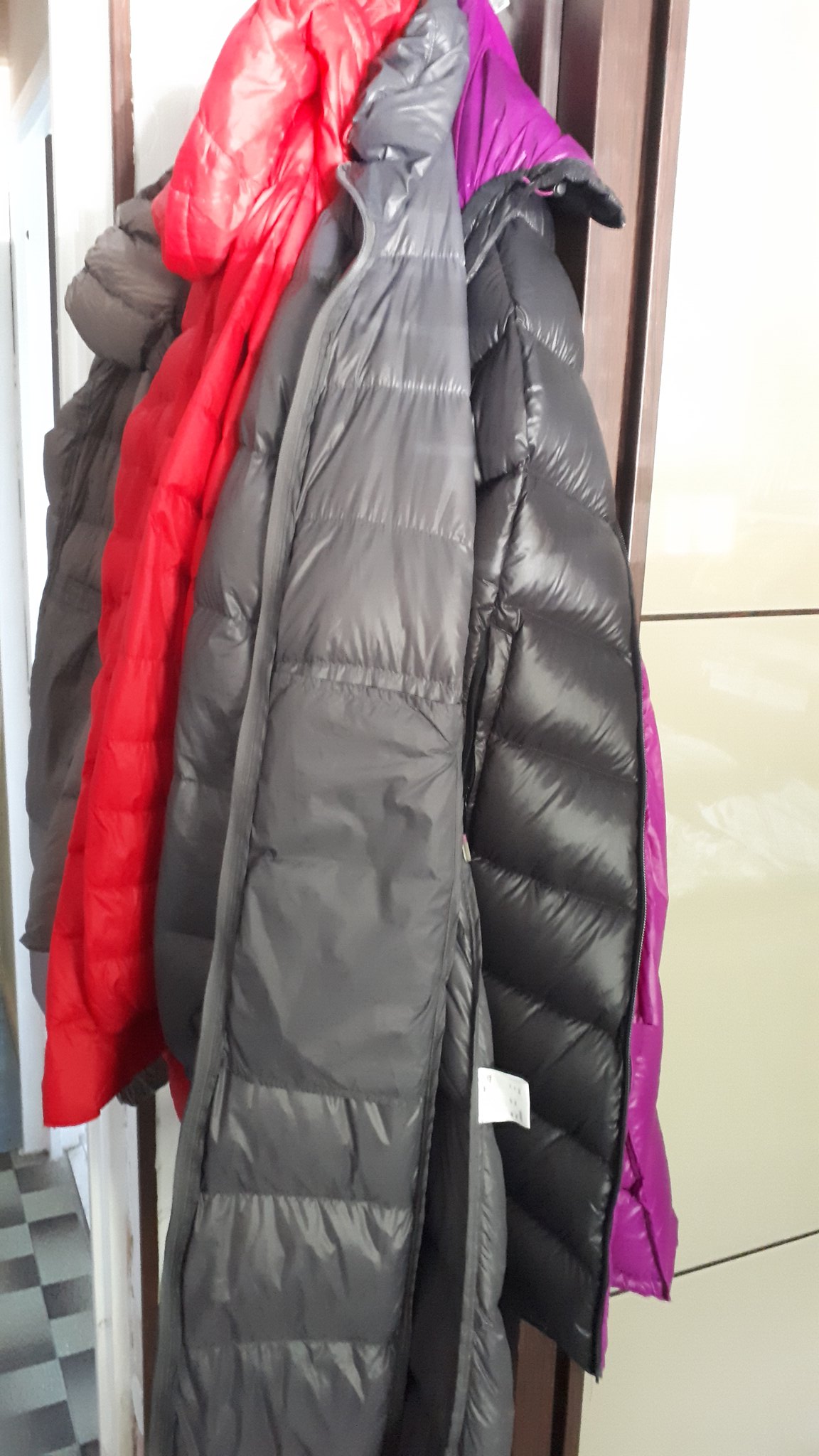This photograph captures two lightweight, puffer-style jackets hanging up. The jacket in the foreground is slate gray with a vivid red lining, while the one in the background is black with a deep purple lining. The jackets are characterized by horizontal seam lines that create a distinct puffed appearance between the seams. The scene is tightly zoomed in, showing minimal background details. On the bottom left, part of a black and gray checker-patterned floor is visible. To the right, a strip or possibly drawers and what looks like large tiles or panels with gray grout lines hint at the surrounding room. The image appears to be taken indoors, possibly in a well-lit area that includes both a floor and a wall.